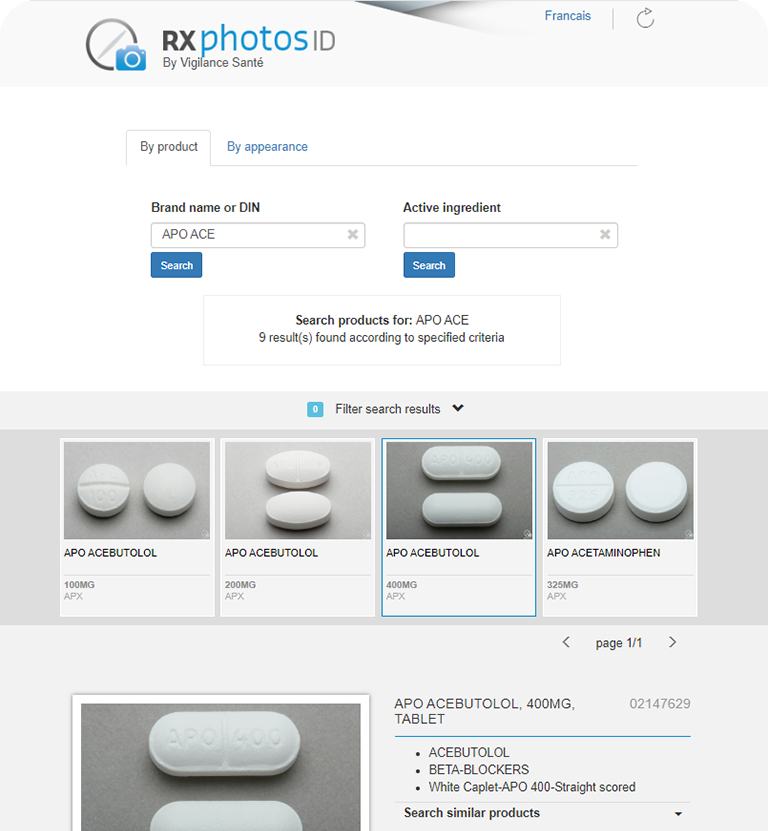The image depicts a webpage from RX Photos ID by Vigilance Santé, a French website currently set to the French language. The website allows users to search for pharmaceutical products either by product name or appearance. The displayed page is the 'by product' search option where users can input a brand name or a Drug Identification Number (DIN) and click on the search button. Similarly, the active ingredient search field allows users to input an ingredient and click on search.

In the example shown, the brand name "A-P-O-A-C-E" has been entered into the search field, yielding nine pharmaceutical drug results containing these letters in their names. The results include a variety of pills with different shapes and dosages: one is a circular pill of 100 milligrams, another is 325 milligrams, and yet another is an oval-shaped pill of 200 milligrams. Each drug result details the pill’s appearance and size. Clicking on any of the images provides an enlarged view along with more detailed information about the product, such as its classification, which might include details like "beta blockers."